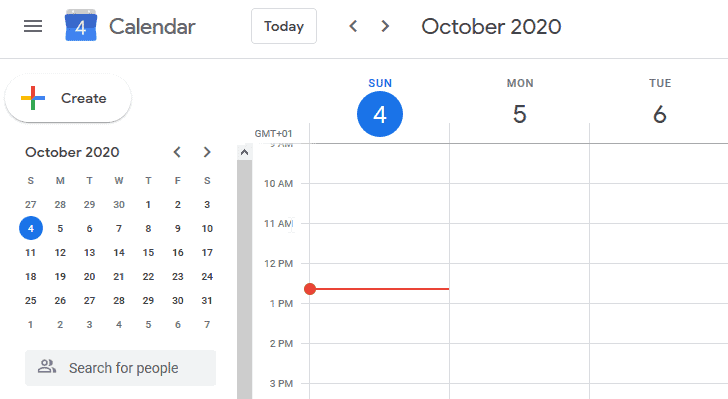The image is a screenshot from the Google Calendar app, specifically highlighting a day in October 2020. A detailed look at the interface shows that the calendar is open to October 4th, which falls on a Sunday. At the top of the image, the date "October 2020" is displayed prominently on the right, with a button symbolized by three black lines in the top left corner for additional app options.

In the main view, there is a clear indicator for Sunday, October 4th, 2020. A red line, connected to a red dot, is visibly marking the time between 12 p.m. and 1 p.m., suggesting an important event or reminder at this time. 

In the bottom left corner, there is a mini-calendar for the entire month of October 2020, where the date 4 is circled in blue, indicating the currently viewed date. Above this mini-calendar, a multi-colored plus sign button (displaying red, blue, green, and yellow) is available for users to create a new agenda or event.